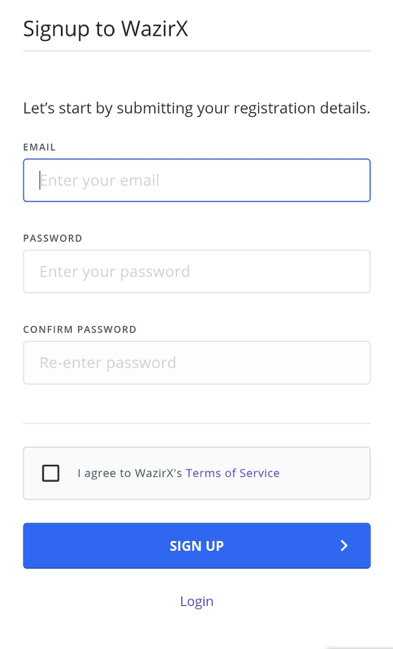The image displays a registration page for WazirX, a cryptocurrency exchange platform. Dominating the center of the interface are fields to enter your email address, create a password, and confirm the password. Beneath these fields, there is a mandatory checkbox labeled "I agree to the terms of service," which, when checked, acknowledges acceptance of WazirX's terms and conditions. A hyperlink is available to review these terms in detail, which will open in a new tab. At the bottom of the sign-up form, a prominent blue button labeled "Sign Up" invites new users to complete their registration, while an alternative "Log In" button is provided for returning users. The minimalistic design and layout suggest this could be a mobile-optimized site. WazirX is clearly branded, with a capital "W" and ending in a capital "X" (W-A-Z-I-R-X). The form seems straightforward, ensuring users confirm their passwords to avoid any typing errors.